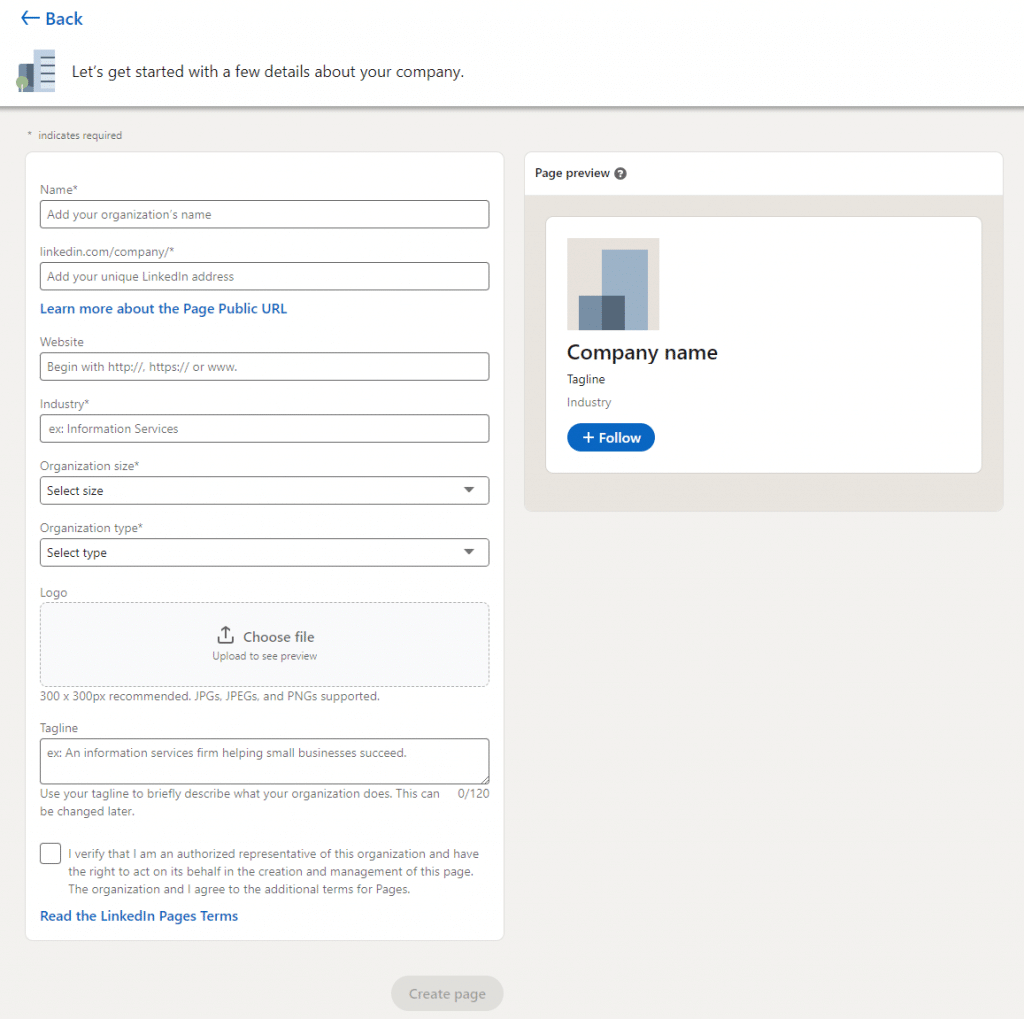The image shows a web page with a form, set against a gray background, designed for users to create a LinkedIn company page. The form itself is white and prominently displayed on the left-hand side of the screen. 

At the top, the form prompts users with "Let's get started with a few details about your company." The first field is for entering the company's name, followed by a field for the organization's LinkedIn URL, highlighted in blue with a "Learn more about Page Public URL" link. 

Next, there is a field to enter the company's website, followed by an industry box where users can specify their industry. An organizational size drop-down menu allows users to select the size of their company. Similarly, an organizational type drop-down menu is provided for users to classify their organization.

The form also includes an option for users to upload the company's logo by clicking on a designated box. Beneath this, there is a tagline section where users can write a brief description of their industry. The instructions for this section remind users to "use your tagline to identify and describe what your organization does."

At the bottom of the form, there are checkboxes for users to verify their status as authorized representatives of their organization. Additionally, there is a link to review LinkedIn page terms. Once all the fields are filled out and the necessary verifications are made, users can click to create their page. At the top of the screen, there is a preview section where users can see what their LinkedIn company page will look like once it’s created.